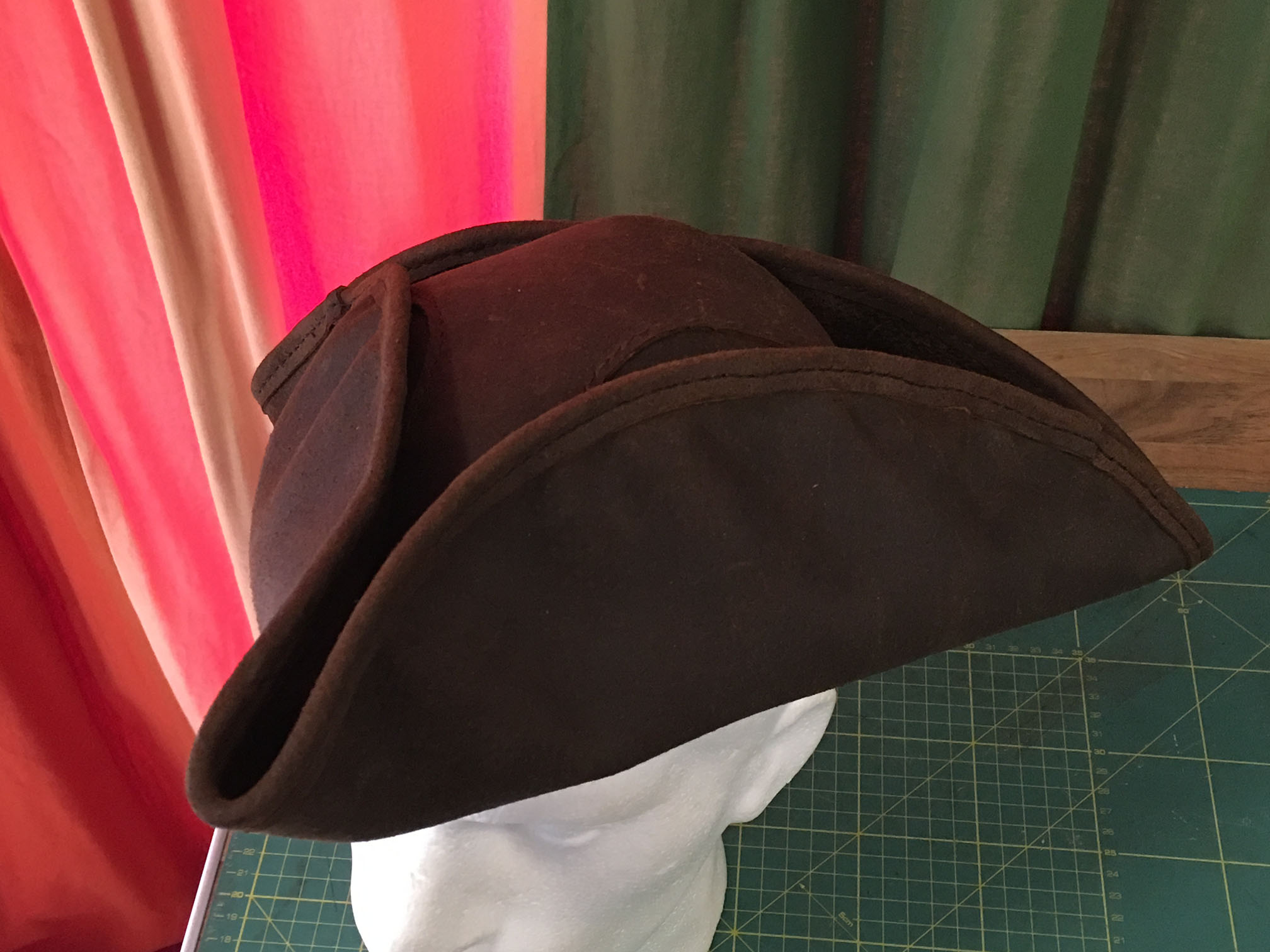The photograph features a white sculptural bust of a face, topped with a deep brown tricorn hat that resembles a pirate's cap. The facial features of the sculpture are somewhat indistinct, particularly around the eyes, which are partially obscured. The bust is set on a green measuring board, designed for accurately cutting cloth. The scene is enriched with green checkered and striped patterns on the table, and the setting includes a wooden floor. A pleated green drapery hangs from the upper right corner, while another drapery in red, pink, and beige tones is visible in the left corner.